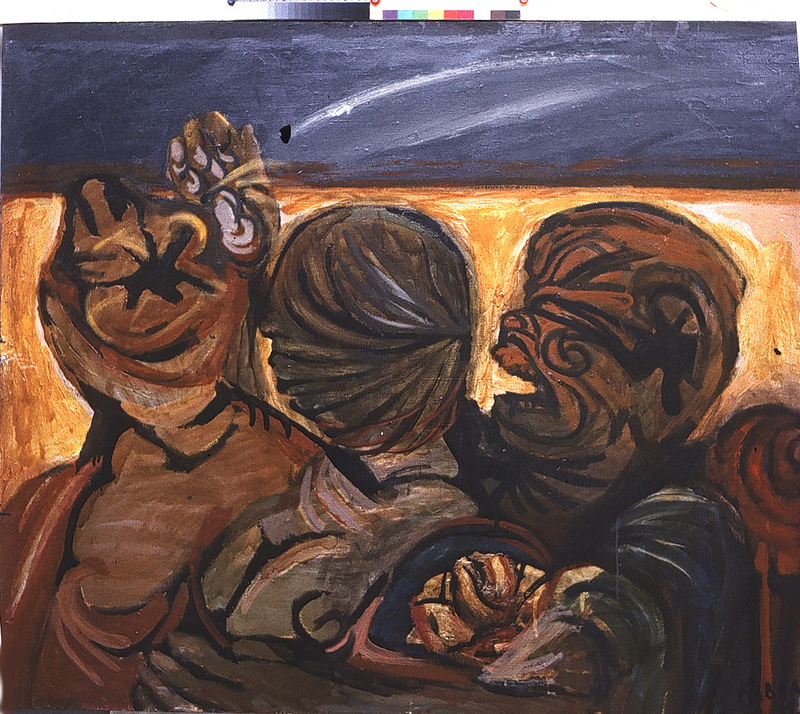In a dark, almost night-time setting, an abstract painting reveals three enigmatic figures in a square-like frame. The top section of the painting depicts a dark blue night sky with streaks of white, transitioning from navy on the left to a lighter blue on the right. Just below, a horizontal line of black and white swatches is paralleled by another line of various colors.

The main composition involves three abstract heads, predominantly brown, positioned in the foreground. The rightmost figure appears distressed, mouth agape as if screaming, and features a mix of black on its head. This figure reaches out with one hand towards a central, ambiguous object, while the other hand seems to hold or interact with the middle figure.

The central figure, resembling a mummy with dark brown swept-back hair, appears to be carrying a bag which holds what might be another head. This figure faces away from the viewer, adding layers of mystery to the scene.

The leftmost figure is characterized by an unidentifiable, possibly masked or disfigured face, holding a notably brown, almost foreboding presence. Together, these abstract characters create a chilling, powerful impression of angst and enigma, evoking multiple interpretations and emotions.